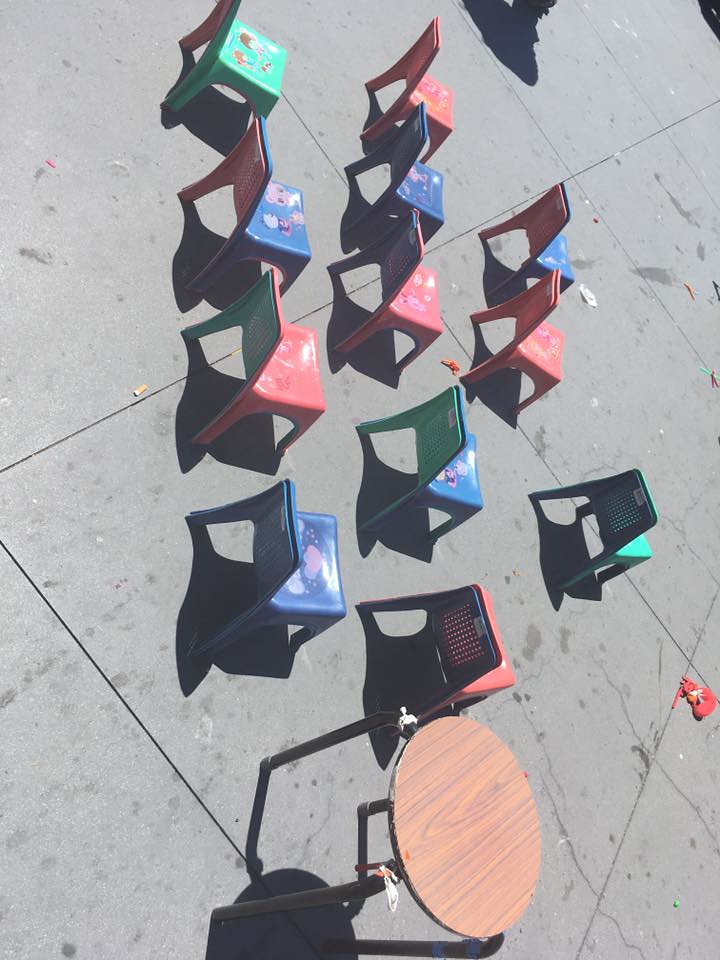This vertical color photograph, which appears to be originally taken horizontally and then flipped, captures a brightly sunlit outdoor scene, possibly a large patio or plaza, at an odd aerial angle. The ground consists of big square cement tiles marred with splotches, marks, stray pieces of trash, cigarette butts, and deflated balloons scattered about. In the image, several small, multicolored plastic chairs in shades of red, blue, and green are arranged in a rough semicircle, all facing toward the right side of the frame. Although some perspectives suggest the chairs might be stacked, upon closer inspection, they are individually placed in three neat rows, casting deep shadows due to the intense sunlight. The chairs, designed for kids, are adorned with various stickers and decals on their backs and seats. Additionally, a small round table with a wood formica top and four metal legs is positioned at the bottom of the image. The photograph's composition and striking brightness reflect a vibrant, albeit slightly chaotic, outdoor setting.